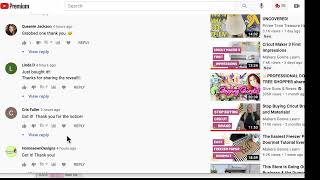**Detailed Caption:**

The image depicts a screenshot of a YouTube video page. At the top left, the distinctive YouTube logo — a red rectangle with a white play button in the center — is clearly visible, signifying the platform. Below the video, four user comments are shown, each accompanied by a profile picture or an initial encapsulated within a circle. The user's name and the time since the comment was posted are displayed next to each comment. 

On the right side of the image, there is a sidebar featuring thumbnails of suggested videos. There are six thumbnails in view, though the sixth thumbnail appears partially cut off at the bottom. Each video thumbnail includes an image representing the video content. Additionally, each suggested video has a small black box in the lower-right corner indicating the video's duration.

At the bottom of the screenshot, a red progress bar spans the width of the screen, hinting at the playback progress of the currently viewed video.